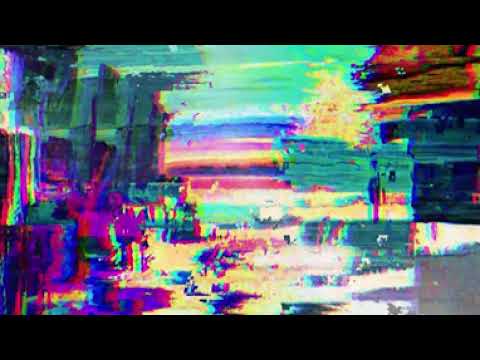The image appears to be an abstract painting with a diverse and vibrant palette, showcasing a mix of colors and strokes. The composition features a variety of hues, including stripes and blobs of purple, blue, dark blue, turquoise, green, bright green, yellow, orange, red, black, and white, creating a visually dynamic piece. The top and bottom sections of the artwork are contained by black areas, framing an array of splashes and rectangles that give the piece a collage-like appearance. The right side predominantly features darker colors such as blues, pinks, browns, grays, and whites. The middle section contrasts with lighter shades including aqua, pink, blue, and some purples, while the left side reverts to darker colors, with an emphasis on blues, pinks, purples, and greens. The bottom left corner is particularly vivid, combining heavy strokes of purple, red, green, and blue. Horizontal lines traverse the middle section, transitioning from green at the top to blue, purple, yellow, dark blue, and red. The lower part of the image features a yellow base with various colored dots that resemble small puddles, accompanied by dark blue and green swirls. The overall effect is almost like a distorted and blocky representation of a canyon or valley, created through an interplay of squares, lines, and brush marks.